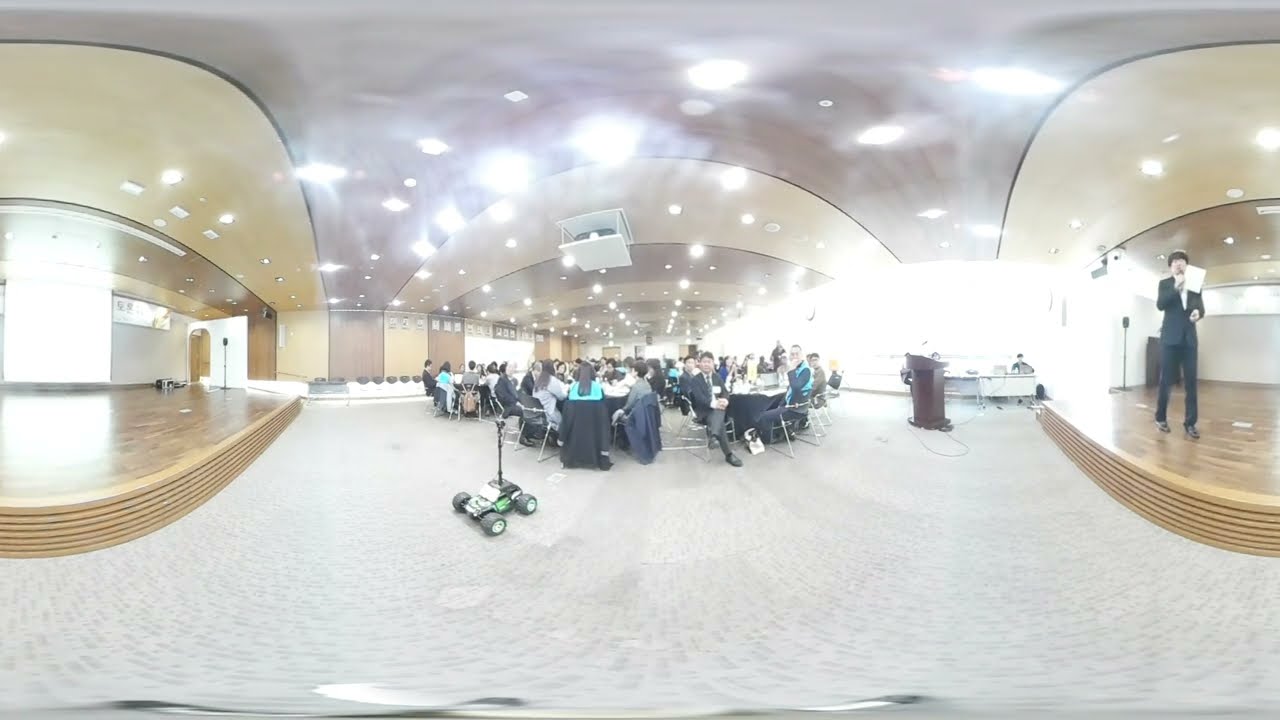This image captures a bustling convention center interior filled with numerous attendees seated at tables. The tables are scattered throughout the center with people sitting on folding chairs, their backs facing the camera, making most faces not clearly visible. Many individuals have jackets draped over their chair backs, hinting at a casual but professional atmosphere. The room is brightly illuminated by several circular light fixtures on the ceiling, casting a strong glow over the entire space. 

On the right side of the image, a man clad in a dark suit stands on a curved wooden stage, his face obscured as he holds a piece of paper or perhaps a phone to his head. Next to this stage, there is a wooden podium with a slanted top, accompanied by a few people sitting at desks nearby. Additionally, in the front center, there is an unusual machine resembling a lawnmower or people mover with four wheels and a handle for steering. The flooring appears to be a mix of gray and beige carpet. The walls and ceiling sport a light beige hue, complementing the overall warm tone of the room. This convention center is a hive of activity, encapsulating the essence of a busy professional gathering.